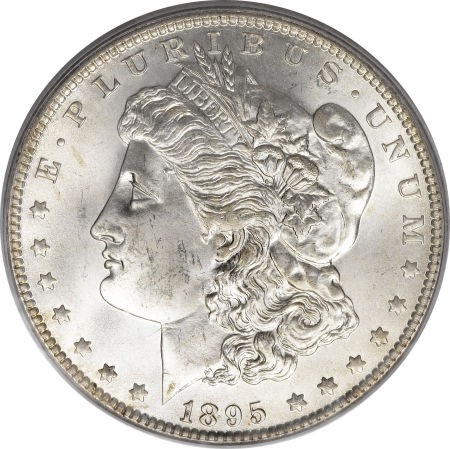The photograph is a close-up image of a silver Liberty Dollar coin, minted in 1895. The coin prominently features the profile of a woman facing left, her hair flowing down her neck. She is adorned with a band in her hair inscribed with the word "Liberty." Surrounding her image, the text reads "E Pluribus Unum" along the upper perimeter, and there are stars circling around. The coin's date, 1895, is clearly visible at the bottom. The image is perfectly centered, providing a clear and detailed view of all the text and design elements, making it appear almost like a stock photo.